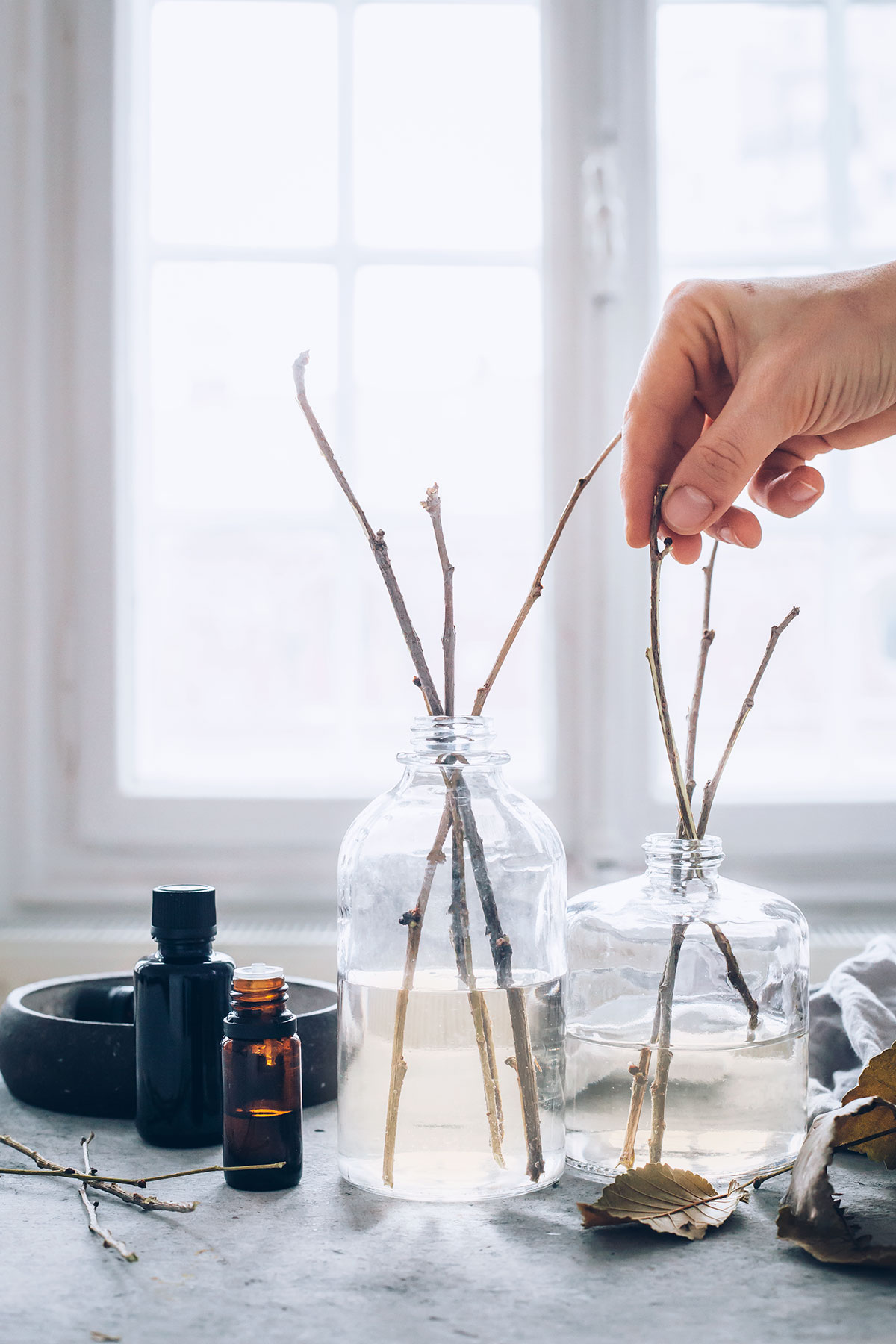This photograph, likely an advertisement for essential oils or natural aroma diffusers, features a serene and minimalist yet sophisticated setting. Centered on a sleek white and gray stone countertop, there are two glass jars filled with liquid—probably infused with essential oils. Each jar contains three rustic wooden twigs, acting as natural diffusers. In front of one jar, a few dried leaves rest, adding to the organic aesthetic. 

To the left of the jars, there are two smaller vials, one black and one brown, with the brown vial’s cap off, suggesting recent use. A hand, belonging to a light-skinned person, is placed delicately inside one of the jars, stirring or positioning one of the twigs. 

In the background, large windows with white frames and a notable white clip on the right window flood the scene with natural light, enhancing the clean and tranquil ambiance of the space. The branches inside the jars are not just simple sticks; they have an authentic, rugged appearance, further emphasizing the natural and eco-friendly theme of the setup.